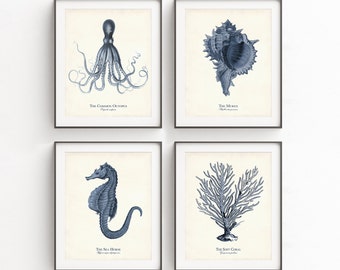This image features four hand-drawn, black and white artworks meticulously arranged in a two-by-two grid on a light gray wall. Each piece is enclosed in a black photo frame, creating a striking contrast against the white matting and tan background of the frames. In the top left frame, there’s a detailed illustration of an octopus with some small, unreadable text below it. Top right features a seashell. The bottom left frame showcases a beautifully rendered seahorse, while the bottom right contains an intricate drawing of a water plant, possibly coral or seaweed. All artworks have accompanying text beneath them, which is too small to discern.